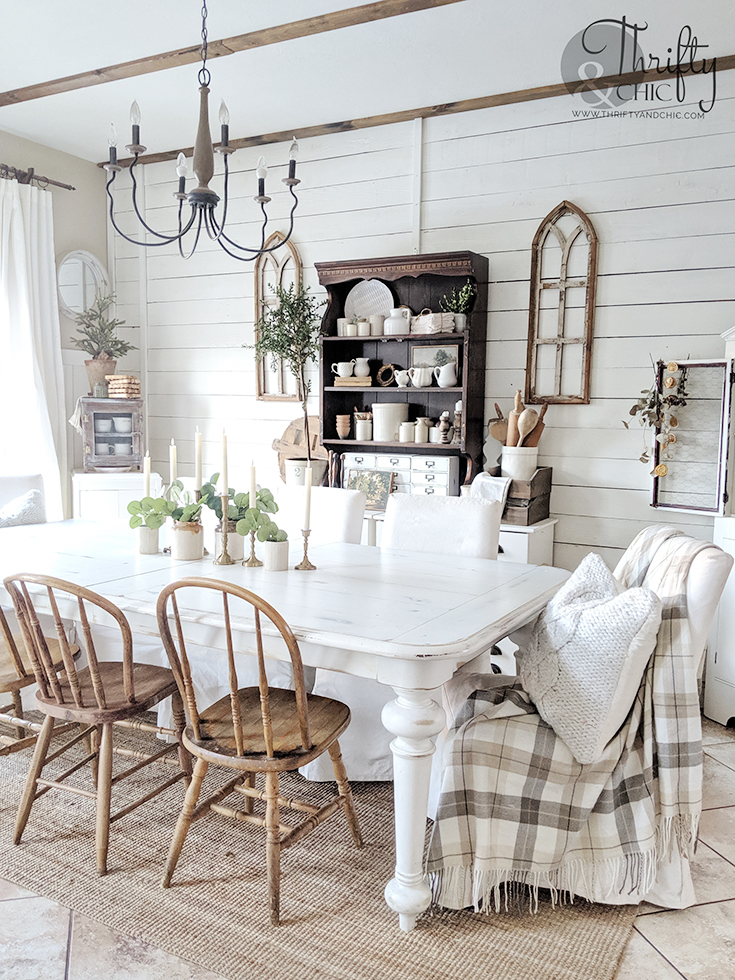The image showcases a pristine dining room characterized by a white theme. At the center of the room is a white wooden dining table, artistically adorned with small potted plants and elegant candles, enhancing the serene ambiance. The photograph is taken from the right-hand side with a slight tilt, emphasizing the single chair at the head of the table. This perspective allows a comprehensive view of the dining table, revealing the back and side walls, both painted in a crisp white color. A graceful chandelier hangs from the ceiling, casting a soft, inviting light over the entire setting, perfecting the room's tranquil and sophisticated atmosphere.